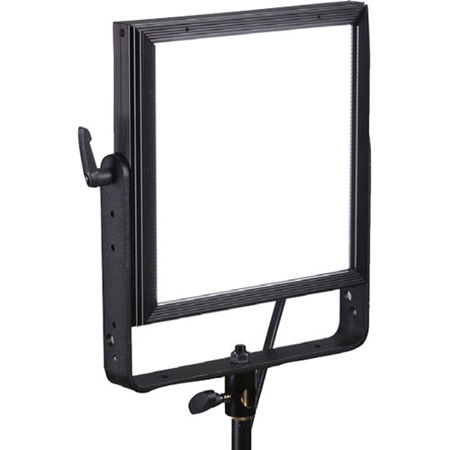The image depicts an apparatus set against a completely white background. Central to the image is a rectangular or square black metal frame. This frame is housed within a U-shaped or horseshoe-shaped black metal housing that includes hand-tightening screws on either side, allowing for adjustments. The middle of the frame is empty, giving the impression that it could be used to look through or to hold another object. The U-shaped housing is mounted on a black metal rod, which itself features an additional hand-tightening screw to secure the base. The apparatus resembles a light stand commonly used in filming, with multiple adjustable screws for modifying its tilt and height. An electrical cord is also faintly visible, suggesting that the device may be powered, although the cord extends out of the frame. Overall, the meticulous arrangement and utilitarian design of the stand, along with its robust adjustment features, hint at its functional role in a professional setting, likely related to lighting or filming.